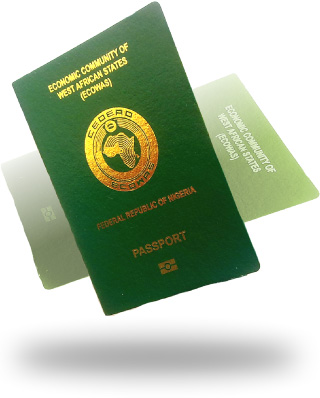The image depicts a green passport from the Federal Republic of Nigeria on a plain white background. The passport is positioned diagonally, with the top angled towards the top left corner. Prominently, it features gold text at the top that reads "Economic Community of West African States" with the acronym "ECOWAS". Below this text, there is a circular gold emblem with the letters "C-E-D-E-A-O" and a gold map of Africa inside a green circle. Further down, the text "Federal Republic of Nigeria" and "passport" is inscribed in gold. Beneath the main passport is a translucent, fainter image of the same passport, oriented diagonally in the opposite direction, creating a sense of depth and a floating effect. Both the primary passport and its shadowy reflection contribute to a visually compelling presentation amidst the stark white background.